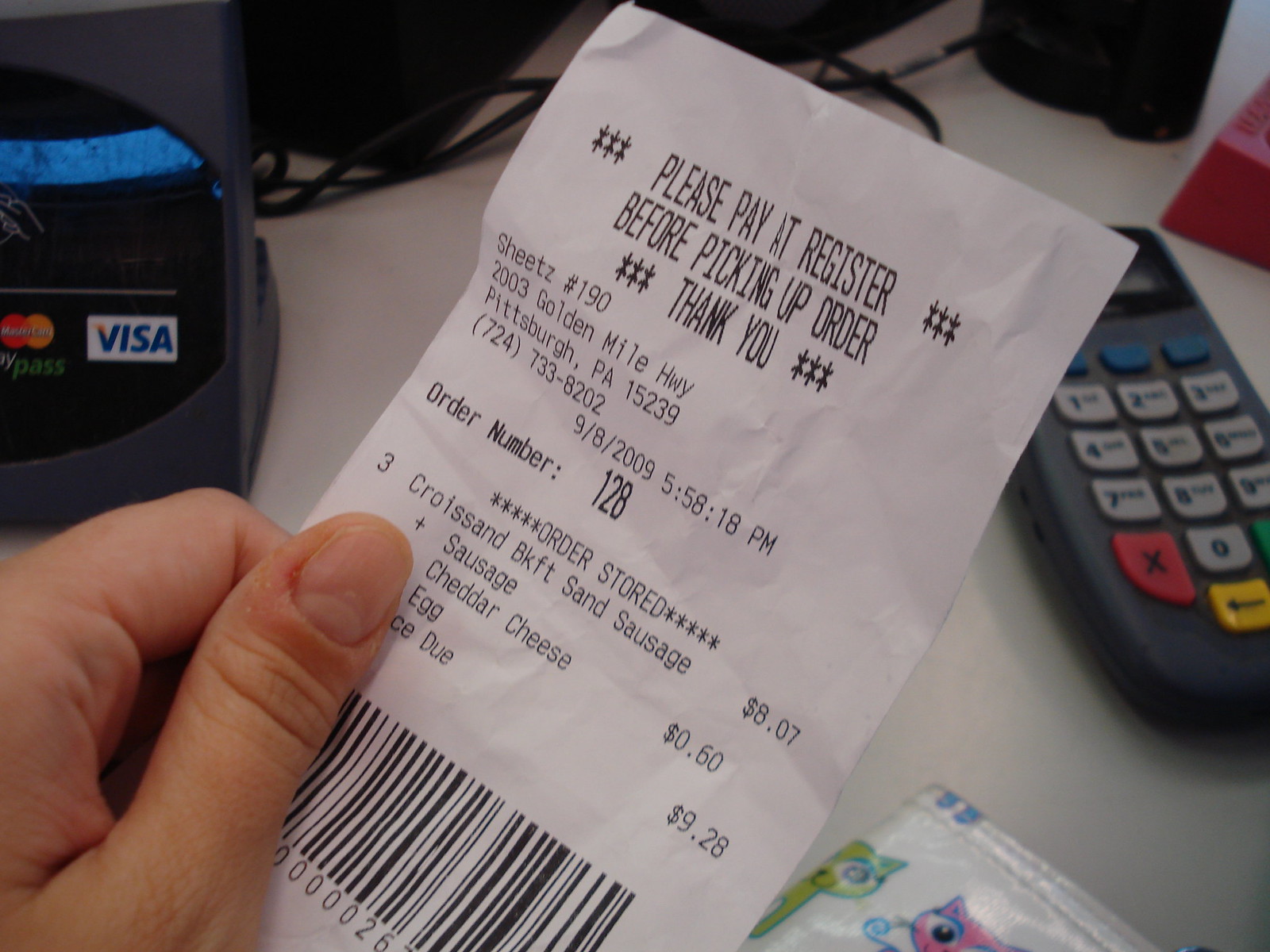The image showcases a detailed view of a receipt held in a man's left hand at a checkout counter. The background features elements of a retail setting, including a partially visible register and card scanner to the left, and a portable fast pay system to the right. The receipt prominently reads, "Please pay at register before picking up order. Thank you." It lists the business name "Sheets #190," located at 2003 Golden Mile Highway, Pittsburgh, PA 15239, and includes a phone number. The transaction took place on 9/8/2009 at 5:58:18 p.m. with an order number of 128. The items detailed on the receipt include a croissant breakfast sandwich and a sausage sandwich with cheddar cheese and egg, totaling $9.28. The barcode is visible towards the bottom.